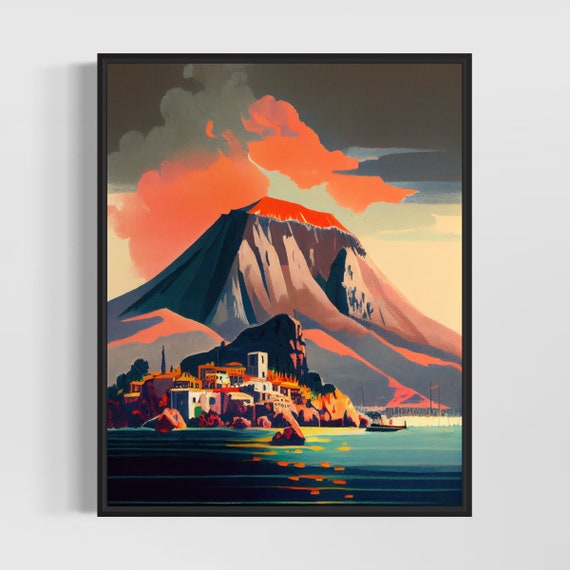The image depicts a striking piece of artwork encased in a thin, black frame, mounted against a white wall. The illustration features a vibrant, erupting volcano. At the peak of the volcano, bright orange and red lava spews into the sky, creating a dramatic contrast against a gradient background that shifts from black at the top to gray and then beige further down. Flowing down the sides of the volcano, the lava path is marked by dark shadows and fiery hues. 

At the volcano's base, a city or village with colorful orange and red rooftops is nestled among rocks that appear almost gorilla-like in shape. The settlement overlooks a body of water, depicted with scattered orange reflections from the volcanic activity. On the water, a solitary boat is visible, situated slightly off-center to the right. Above the village, clouds of orange and gray smoke billow from the eruption, adding to the scene's dynamic and dramatic nature. The entire artwork is clear and vivid, emphasizing the vibrant and chaotic beauty of the erupting volcano.